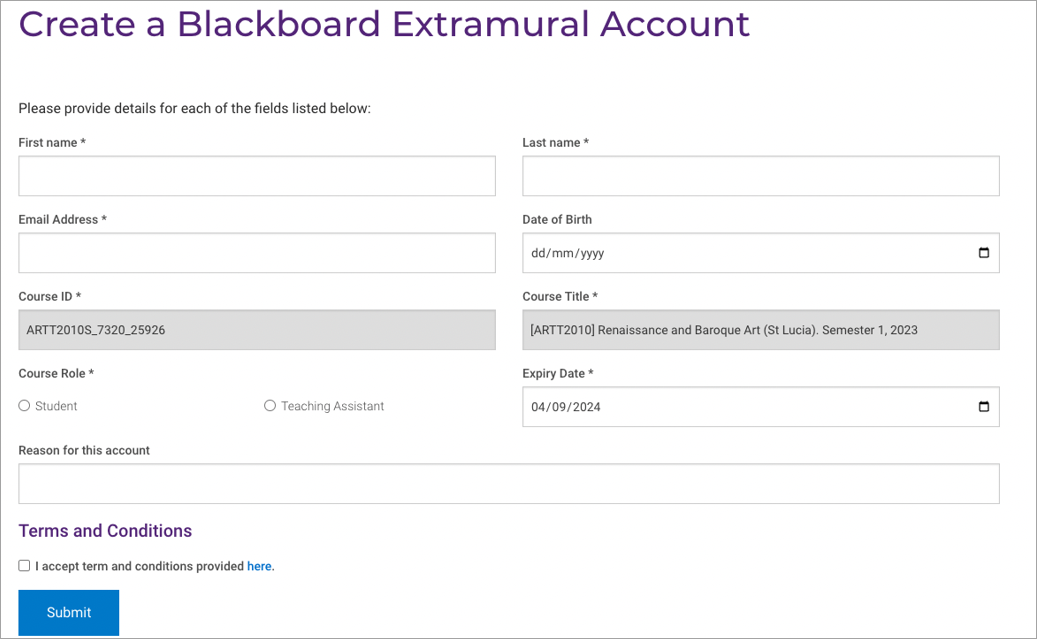The image depicts a registration form for creating a Blackboard extramural account. The form is contained within a white rectangle bordered in grey. At the top left corner, the heading "Create a Blackboard Extramural Account" is prominently displayed in purple. Below the heading, a black instruction prompts users: "Please provide details for each of the fields listed below."

The form includes several labeled fields, many marked with a red asterisk indicating that they are required:

1. **First Name*:** A grey-outlined rectangular input box.
2. **Last Name*:** Another similar grey-outlined rectangular input box.
3. **Email Address*:** A grey-outlined rectangular input box.
4. **Date of Birth:** A grey-outlined input box denoted by the placeholder "DD/MM/YYYY" with a small calendar icon on the right for date selection.
5. **Course ID*:** A grey-outlined rectangular input box already filled with a mix of letters.
6. **Course Title:** A grey-outlined rectangular input box containing letters.
7. **Course Role*:** Contains two options, each accompanied by a circular radio button: 
   - Student
   - Teaching Assistant
8. **Expiry Date*:** A grey-outlined input box featuring a calendar icon on the right for easy date selection.
9. **Reason for this Account:** A long grey-outlined rectangular input box for additional information.

Towards the bottom of the form, "Terms and Conditions" is highlighted in purple. Beside it is a grey-outlined square check-box labeled "I accept the terms and conditions provided."

Finally, at the bottom of the form, there is a blue rectangular button labeled "Submit" in white text, ready for initiating the submission process.